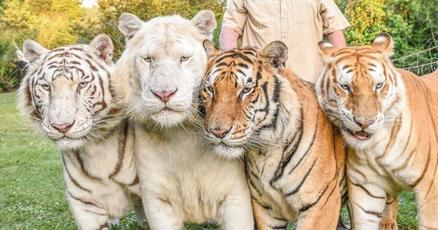In this captivating outdoor image, a man in a pale yellow short-sleeved shirt stands behind four majestic tigers positioned on a lush green grass lawn under the sunny sky. The tigers create an intriguing visual composition with their heads touching, showcasing an array of colors and patterns. On the far left, a magnificent Siberian tiger with light fur and subtle brownish stripes stands next to an almost pure white tiger with barely noticeable stripes. To their right, two typical orange-and-black-striped tigers complete the quartet, one featuring striking blue eyes. The photograph focuses on their heads, chests, and part of their front legs, highlighting their impressive stature and adult size. Surrounding the scene is a backdrop of dark green trees, some tinged with pale yellow at the top, adding to the idyllic natural setting. A section of a fence is also visible behind the group.